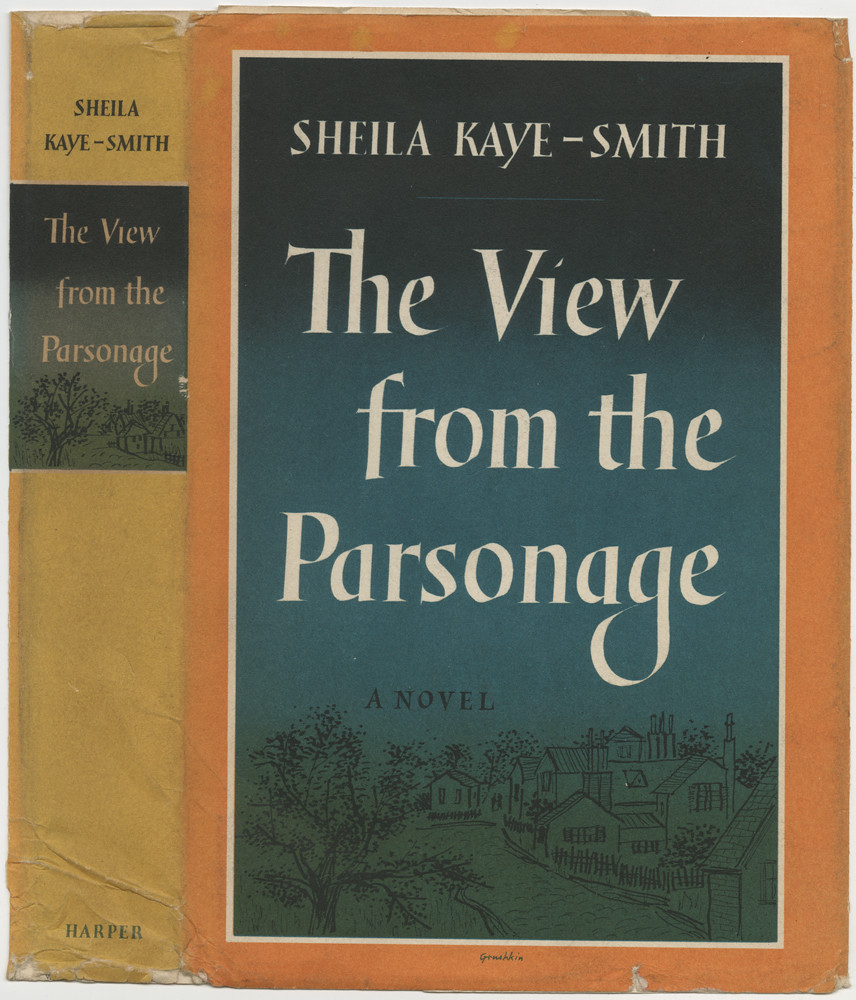The image showcases an older novel titled "A View from the Parsonage" by Sheila K. Smith. The book's cover features a prominent orange border and white text set against a black background. The title, "A View from the Parsonage," is centered and arranged from left to right. The author’s name, "Sheila K. Smith," is also displayed clearly. The book has a yellow spine, adding a contrasting touch to its visual appeal. The cover shows signs of wear, with visible wrinkles and fading, indicating that the book has been well-read and possibly passed down through generations. The book is positioned flat on an indistinguishable surface, surrounded by a plain white backdrop.